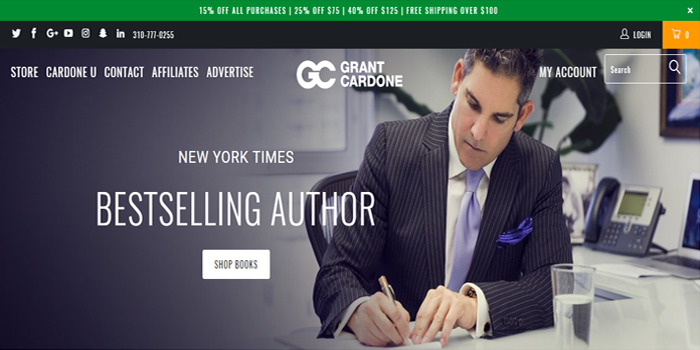This image is a promotional screenshot with several key elements. At the very top, a vibrant green bar displays various discount offers: "15% off all purchases," "25% off $75," "40% off $125," and "Free shipping over $100," along with an 'X' button in the top right corner for closing the banner. Below this, a social media toolbar appears, featuring logos for Twitter, Facebook, Google+, YouTube, Instagram, Snapchat, and LinkedIn, along with the phone number 310-777-0255. 

In the top right section, there are prominently displayed orange-colored buttons for "Login" and "Cart." Beneath this, a navigation bar provides links to "Store," "Cardone," "You," "Contact," "Affiliates," and "Advertise." Central to the header is the GC logo representing "Grant Cardone." Adjacent to this, on the right, is an "Account" button and a search bar.

The background showcases a professional image: a man in a suit within an office setting, intently writing something down. Superimposed on this background, bold text announces "New York Times Best Selling Offer," accompanied by a white button with black text labeled "Shop Books."